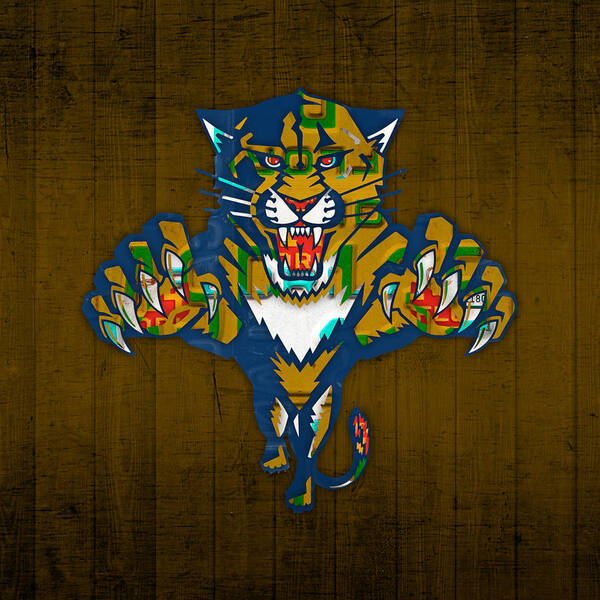This image features a digitally created, vibrant tiger mascot, likely serving as a logo for a school or sports team. The tiger, depicted in dynamic motion as if lunging forward, is adorned with an array of vivid colors: its primary orangish-brown fur is accented with blue, green, and red. Its fierce eyes, nose, and the inside of its mouth are red, while its claws, extended threateningly, have red on the palms. The tip of its curled tail showcases both orange and yellow hues. The background consists of artificially rendered wood paneling in a dark, brown tone, creating a striking contrast to the colorful tiger and emphasizing its central position in the image. The wood panels, though detailed to resemble stained wood, maintain an artificial appearance, highlighting the digital nature of the artwork.